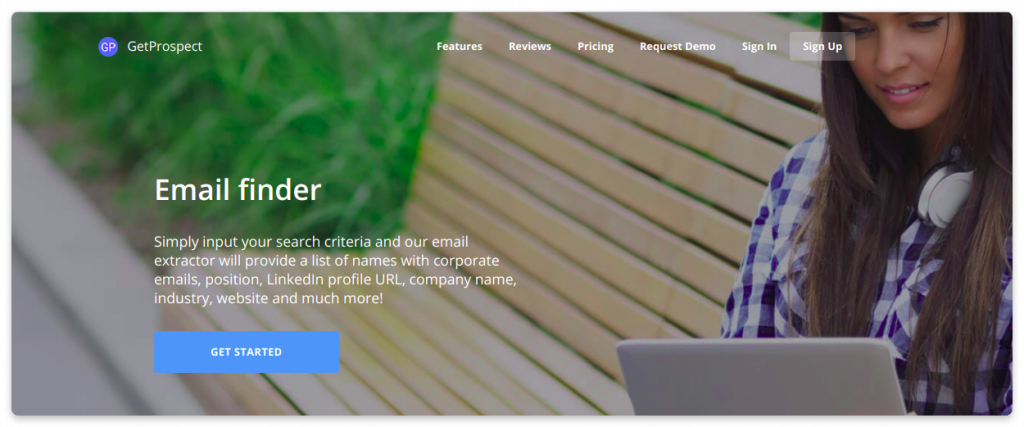The landing page for the "GetProspect" website features a prominent logo consisting of the initials "GP" in white, enclosed within a blue circle. The company's name, "GetProspect," is displayed with capitalized "G" and "P." The navigational menu at the top includes buttons for "Features," "Reviews," "Pricing," "Request Demo," and "Sign In," along with a prominently highlighted "Sign Up" button in white text. Below the menu, the heading "Email Finder" is presented in a larger font with a capital "E" in white text. This is followed by a brief description: "Simply input your search criteria and our email extractor will provide a list of names with corporate emails, position, LinkedIn profile URL, company name, industry, website, and much more." 

A blue "Get Started" button is situated beneath this text. The cover image on the page depicts a woman sitting on a park bench, wearing a scarf, and working on a silver laptop. She has long brown hair and appears to be concentrating on her screen, with her gaze directed downward. The environment includes a bit of grass visible in the upper left corner of the image.